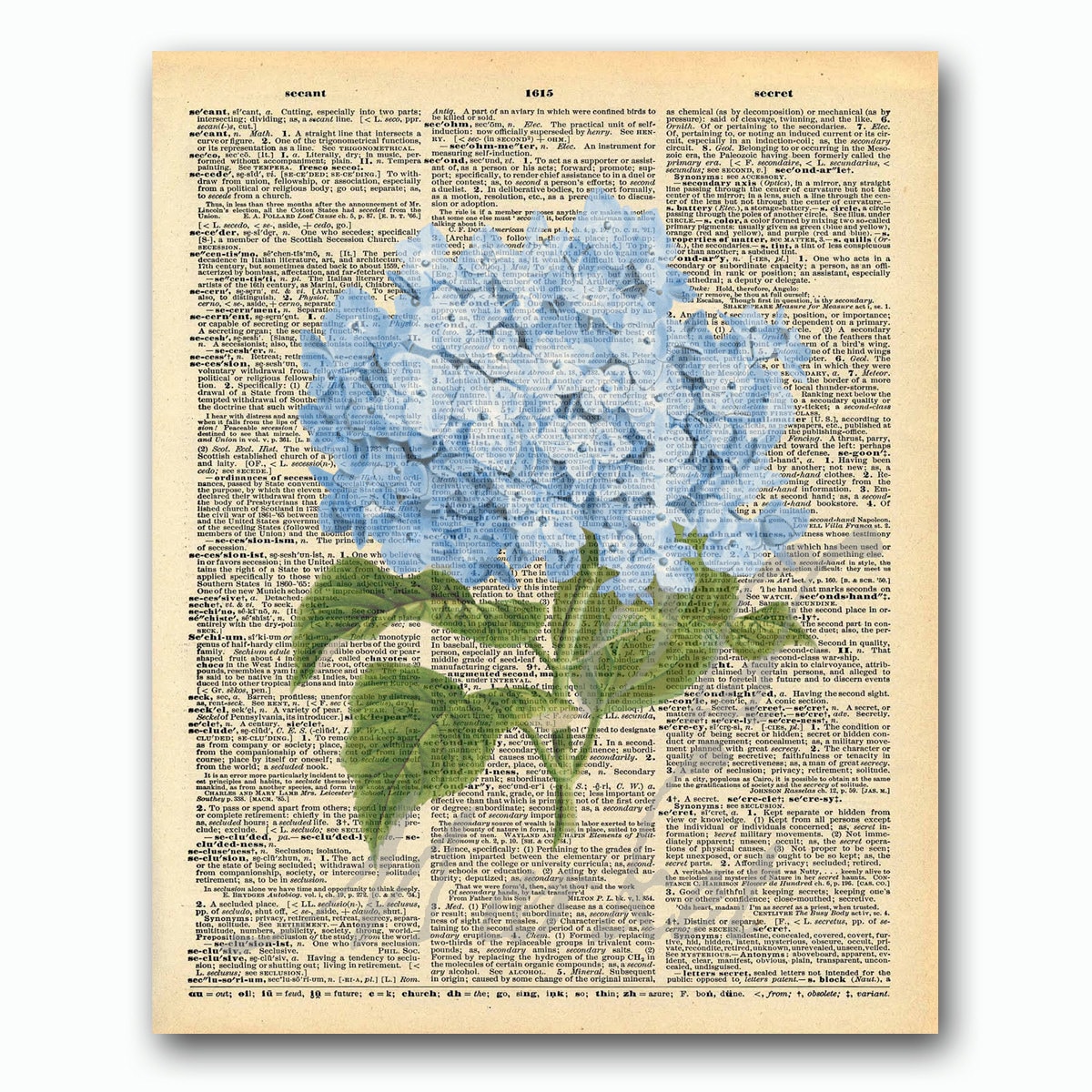The image portrays a page from an old dictionary, displaying an aged, yellowed parchment background with black text organized into three columns of tiny definitions. Topped by the number 1615 at the center, this vintage publication has black, slightly darkened text indicative of its age. Superimposed in the middle is a semi-transparent watercolor illustration of a hydrangea blossom. The hydrangea features numerous blue petals clustered together, accompanied by lush green leaves reaching out in different directions from its stem. The transparency of the illustration allows the underlying dictionary text to be seen through the floral design, adding a layered complexity to the visual experience. The word "MARKET" can be faintly seen in gray text at the bottom, blending seamlessly with the aged aesthetic. The artwork exemplifies a blend of photographic representationalism and vintage print, combining the beauty of traditional dictionary pages with the vividness of floral illustration.